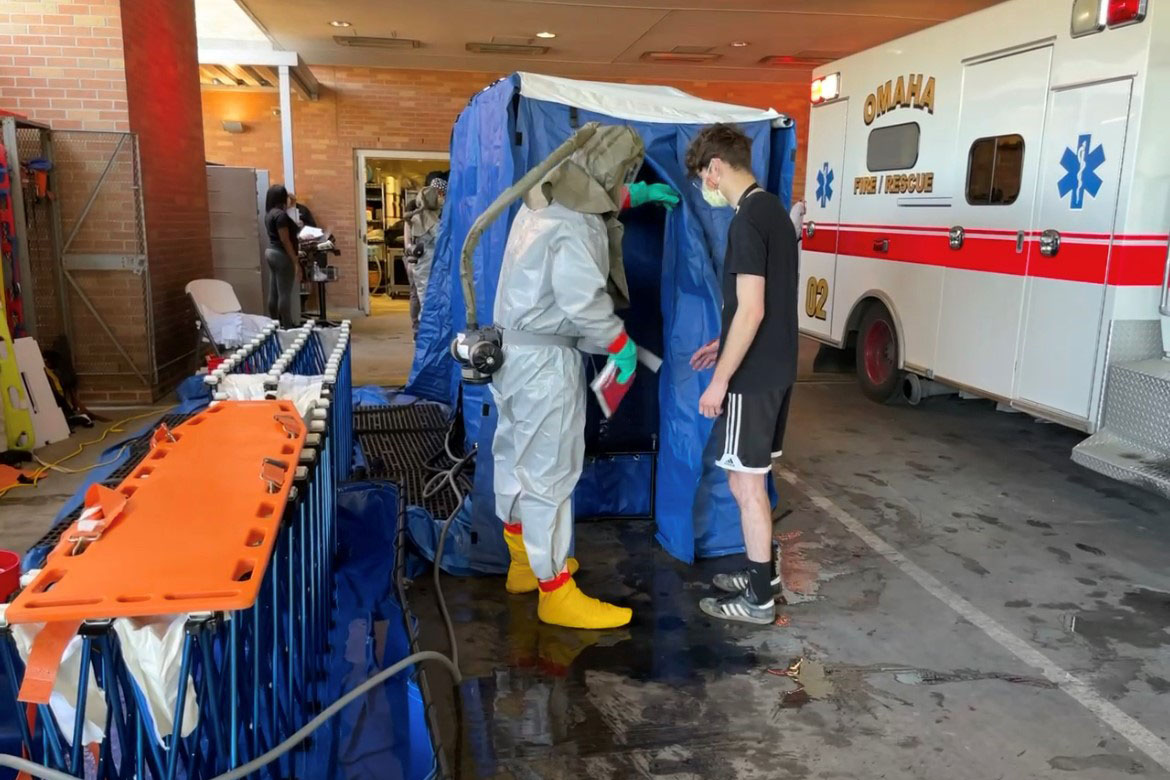This color photograph depicts an emergency ambulance bay adjacent to a hospital, characterized by a broad cement parkway and the brown brick walls of the hospital in the background. Overhead, fluorescent lights illuminate the scene. Dominating the right side of the image is a white ambulance adorned with a red stripe and emblazoned with "Omaha Fire Rescue" and two blue star symbols indicative of emergency medical services.

To the left stands a rectangular blue pop-up tent, possibly serving as a decontamination or triage area. In the foreground, a person dressed in a comprehensive hazmat suit—consisting of a white coverall, yellow plastic boot covers, teal blue gloves, and a ventilator system running from a dark gray hood to a black oxygen tank on their back—holds open the flap of the tent. Just outside the tent, a young male, identifiable by his brown hair and attire including a white face mask, black t-shirt, black shorts, black socks, and black tennis shoes, appears to be about to enter.

The overall scene suggests a hazardous material drill or a real-life decontamination scenario, with the appropriate measures and equipment in place to protect those involved.